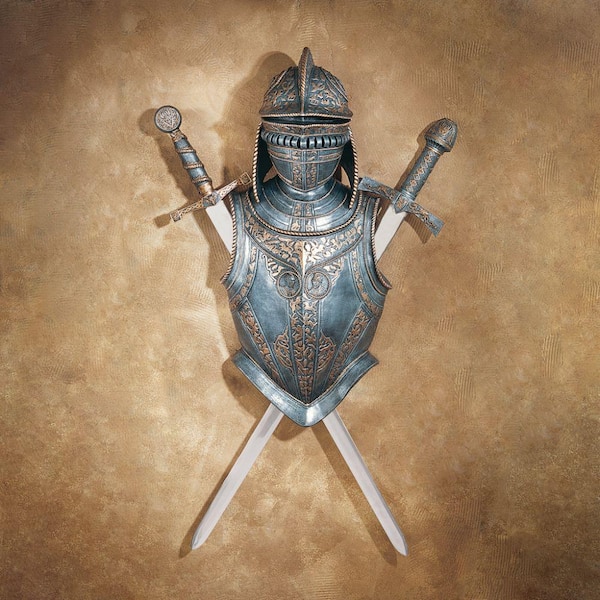This photograph captures an intricate display of medieval knight armor and swords mounted on a light brown, stucco-like wall. Centered in the image is a detailed dark gray chest plate adorned with gold and bronze filigree, featuring a V-shaped band that runs from the bottom left, curves down to the middle, and ascends back to the right. Positioned above the armor is a helm with a pronounced ridge running down the center, coiled details beneath a horizontal eye slit, and protective flaps edging the sides, accentuated with golden highlights.

Flanking the helmet and integrated into the armor itself are two swords, their handles protruding outward. The sword on the left has a round end at the handle, and the one on the right features a dome-shaped handle. Both blades enter through the armholes of the chest plate and cross in an X-shaped pattern behind the armor, emerging again at the bottom. The sword handles carry a similar dark gray aesthetic, complemented by blue and gold or copper decorations. A soft, glowing light casts from the center, enhancing the beige hue of the wall and enriching the overall visual allure of this medieval ensemble.